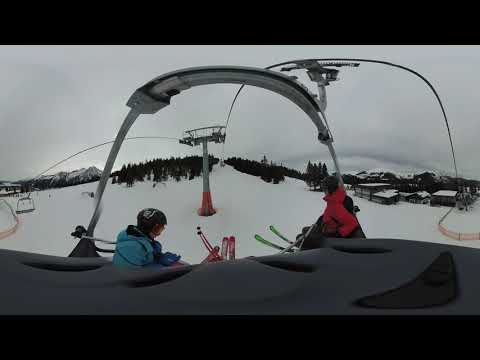This photograph captures a daytime winter scene at an outdoor ski resort, featuring two people seated on a ski lift. The person on the left is wearing a light blue jacket, a black helmet, blue gloves, orange reflective goggles, and has red skis and ski poles. Next to them, on the right, is another person in a red and black jacket, a black helmet, black-rimmed goggles, and green skis. They both appear to be looking in different directions, one slightly down and the other slightly up.

The setting is characterized by thick snow covering the terrain, a gray and cloudy sky, and distant snow-capped mountains with a green tree line. The ski lift is mechanically operated, consisting of multiple wires attached to large silver pillars with orange pads at the base and crossing arms supporting the wires. The black seats of the ski lift stand out against the snowy backdrop. Additional details include metal poles indicating the structure of the lift and buildings covered in snow, located down a slope to the far right. The wide-angle lens used for this photograph creates a slightly distorted, curved appearance of the ski lift, capturing the expansive outdoor environment on this dull, hazy day.